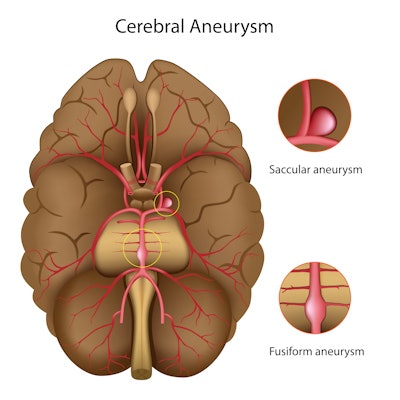The image is a detailed, textbook-style medical illustration of a brain with cerebral aneurysms. At the top, the title "Cerebral Aneurysm" is prominently displayed in black letters against a white background. The main drawing on the left side of the image depicts the underside of a human brain, presented in light brown with segments outlined in a bone-white color. Red veins branch out from the center divider, adding a sponge-like texture to the brain. A yellowish-gold base of the skull is visible at the bottom. Highlighted within the brain is a pink dot circled in yellow, indicating a specific aneurysm.

To the right are two smaller, circular insets. The upper circle features a red vein with a balloon-like protrusion, labeled "Saccular Aneurysm" in black text. This depiction resembles a pink bud on a brown background. The lower circle shows another red vein, this one extending vertically and bulging outward at the base, labeled "Fusiform Aneurysm." This provides a clear contrast between the two types of aneurysms, effectively illustrating their differences.